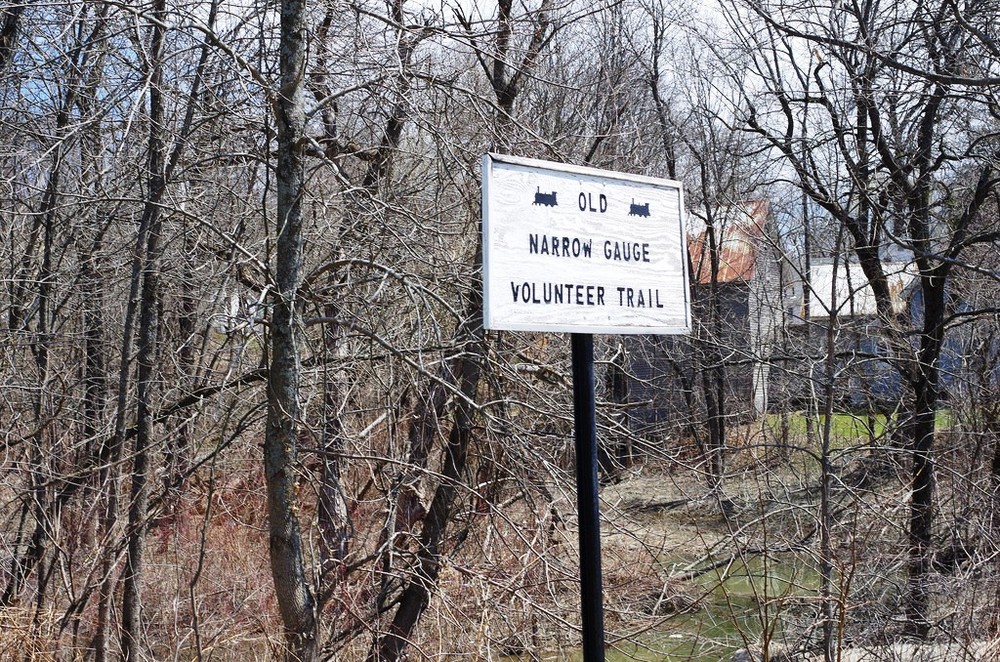A white, rectangular sign faces right, situated amidst a scenery dotted with leafless trees. The background to the left is predominantly occupied by tall trees with thick trunks, their ends disappearing out of frame, while the right side features a shorter tree with a visible split, its top slightly peeking out amidst branches. The sign itself has three rows of text in all capital letters: "OLD" at the top, flanked by images resembling the front of a train locomotive, "NARROW GAUGE" in the middle, and "VOLUNTEER TRAIL" at the bottom. To the right of the sign and left of the shorter tree, a cluster of old buildings with dark gray walls and red and white roofs adds to the rustic charm of the scene.